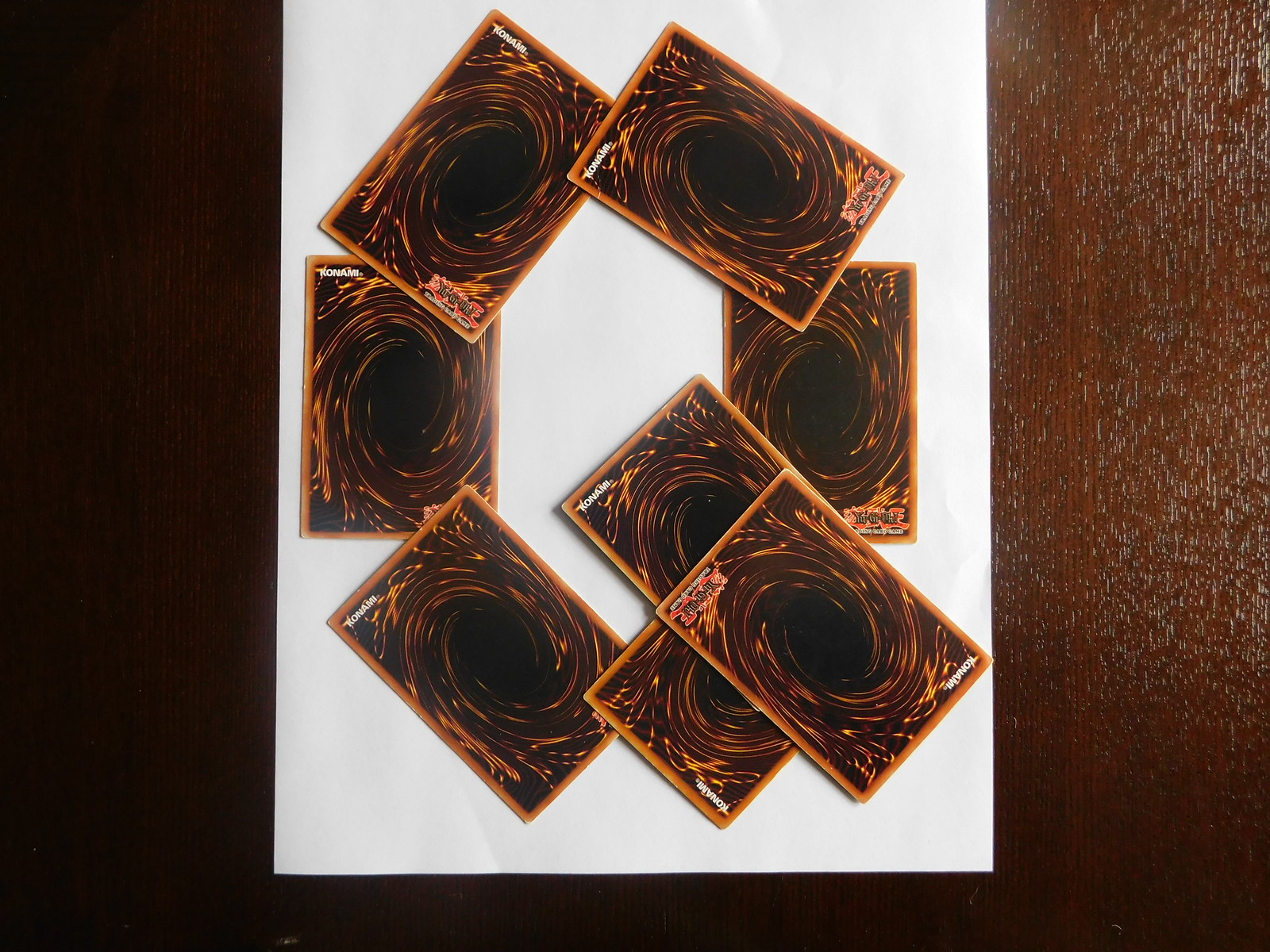This photograph showcases a collection of approximately ten Yu-Gi-Oh! trading cards, arranged in a circular formation on a standard 8.5 by 11-inch sheet of paper. The cards are all placed face down, obscuring their detailed faces from view. 

The surface beneath the paper appears dark and challenging to discern, although there are hints of wood grain, suggesting a wooden tabletop as the underlying material. The cards themselves are decorated with intricate, fiery swirls in a spectrum of colors, all converging towards a deep black center. The borders of the cards are a striking gold-orange hue, adding a vivid contrast to the swirled backgrounds. The dimensions of each card seem to be approximately 3 by 2 inches. The overall composition creates a mysterious and dynamic visual effect, emphasizing the rich detailing characteristic of Yu-Gi-Oh! cards.